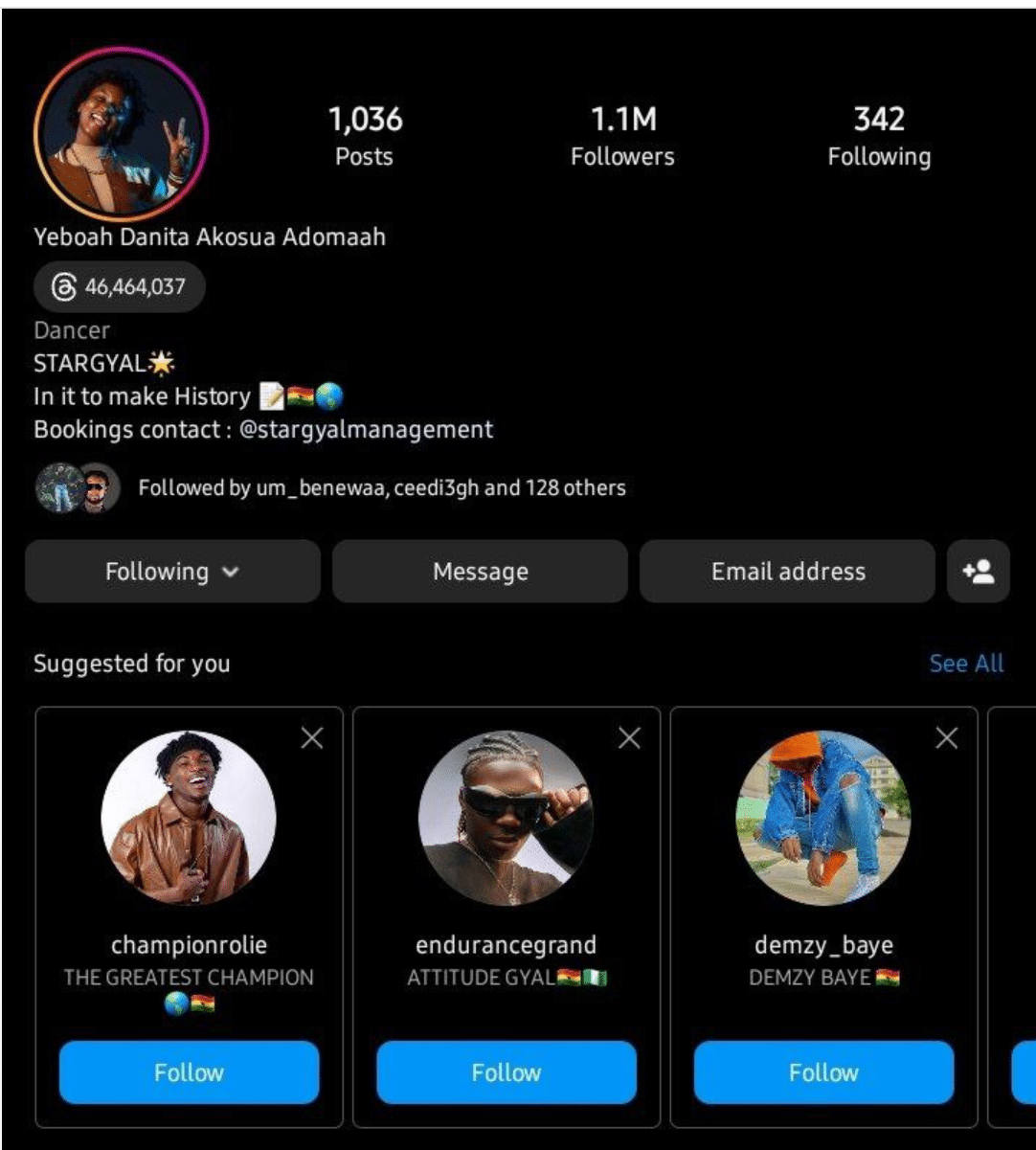This vertical image, seemingly captured from a smart device, portrays a social media profile interface against a solid, jet-black background. In the top left corner, there’s a profile picture enclosed in a partial ring of purple and orangish-yellow. Positioned next to the profile picture, the text displays: "1,336 posts, 1.1 million followers, and 342 following."

The profile name is stated clearly as "Yeboah Danita Akasua Adoma," followed by her descriptive tagline: "Dancer, star gal, in it to make history." Additionally, it mentions details for bookings and lists some followers.

Interactive buttons such as "Following," "Message," "Email," and "Add Friend" are readily available. Below these details, there’s a "Suggested for you" section on the left side, with a "See All" button on the far right. This section features three vertical images of different users alongside their names, with options to "Follow" or dismiss them by clicking an "X."